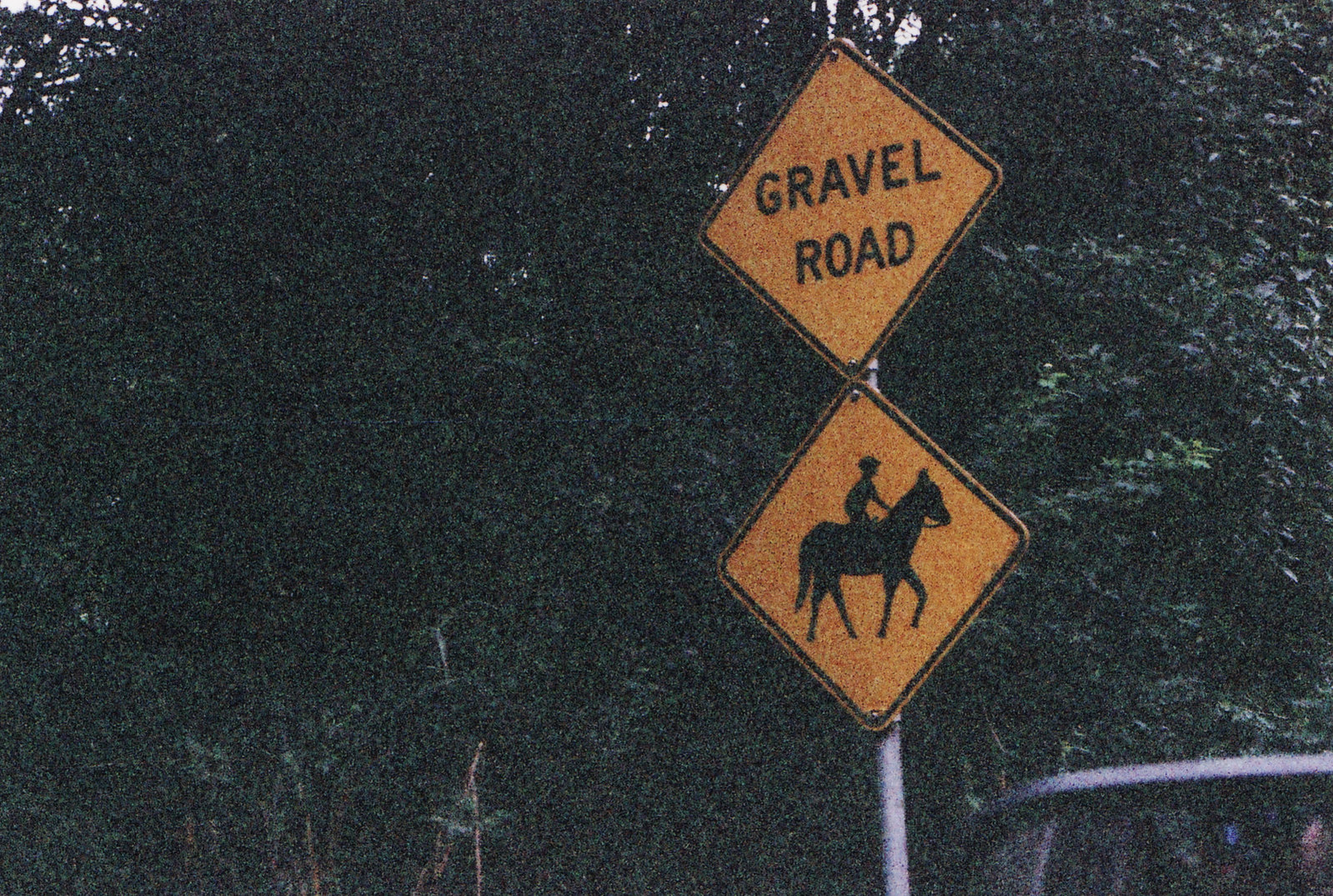The image depicts a fairly grainy scene of a gravel road, hinting at an equestrian school or simply an area where horseback riding is common. The focus points are a horse carrying a young boy, set against a backdrop of a tree line. A car's side mirror occupies the right side of the image, indicating it was taken from the driver's side window. Despite the graininess, green vegetation and standard yellow road signs are discernible throughout the shot. The reflection in the mirror is indistinguishable, adding to the overall enigmatic feel of the night-time photograph.